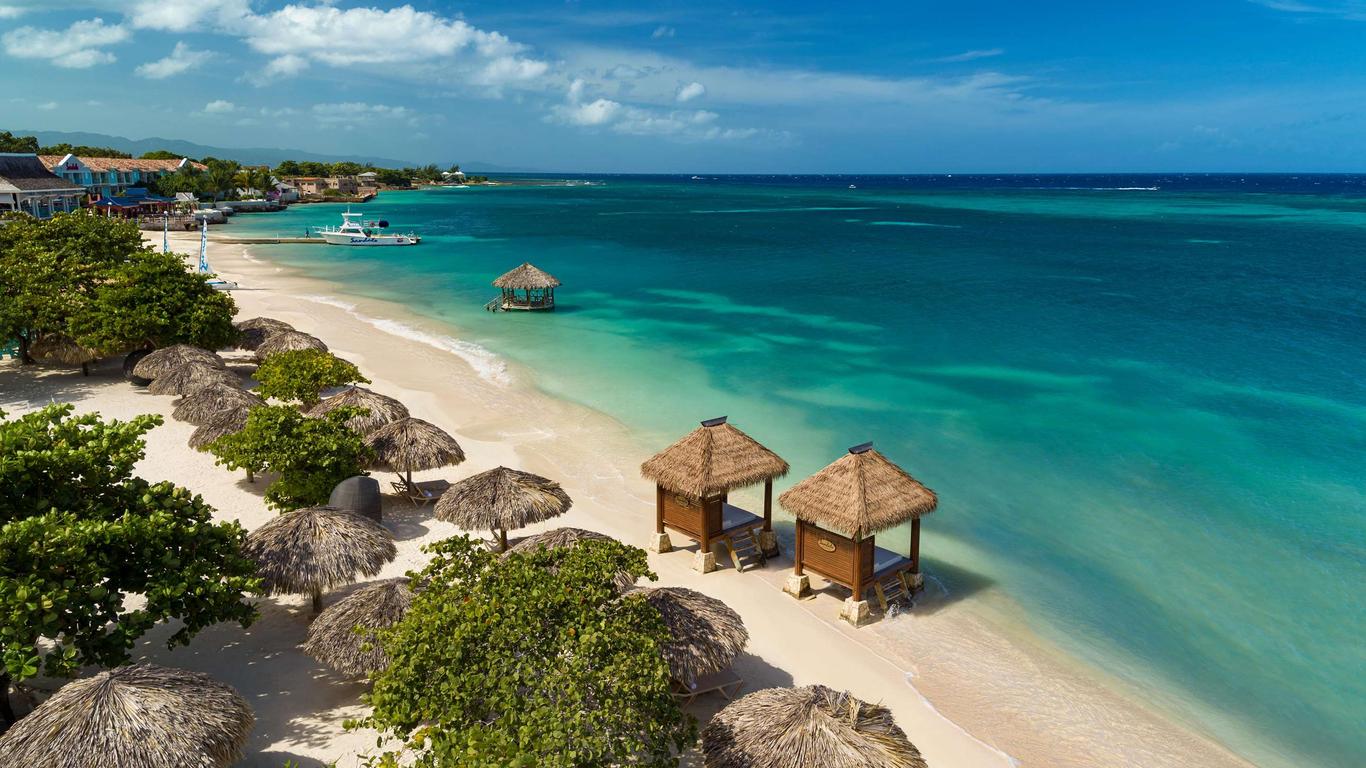This image captures an aerial view of a pristine tropical beach resort, likely situated in the South Seas. The crystal-clear ocean spans the right side of the image, transitioning from a greenish hue near the shore to a deeper blue further out. The beach itself is composed of light, clean sand with no visible people. 

Dotting the shoreline are various rustic, primitive-made umbrellas crafted from sticks or straw, under some of which chairs are neatly arranged. There are small huts, some set directly in the water and others on the beach, along with walkways connecting them. In the distance, a white boat is seen to the left, moored near a wooden dock. 

The sky above is a mostly clear blue with some scattered clouds on the left side. Lush green trees frame parts of the beach, adding to the tropical ambiance. The resort area is lined with what appears to be large houses or hotels, providing a luxurious backdrop to this serene landscape. The colors are vivid and diverse, including hues of blue, green, white, brown, and even touches of red, capturing the vibrant and tranquil essence of this tropical paradise.